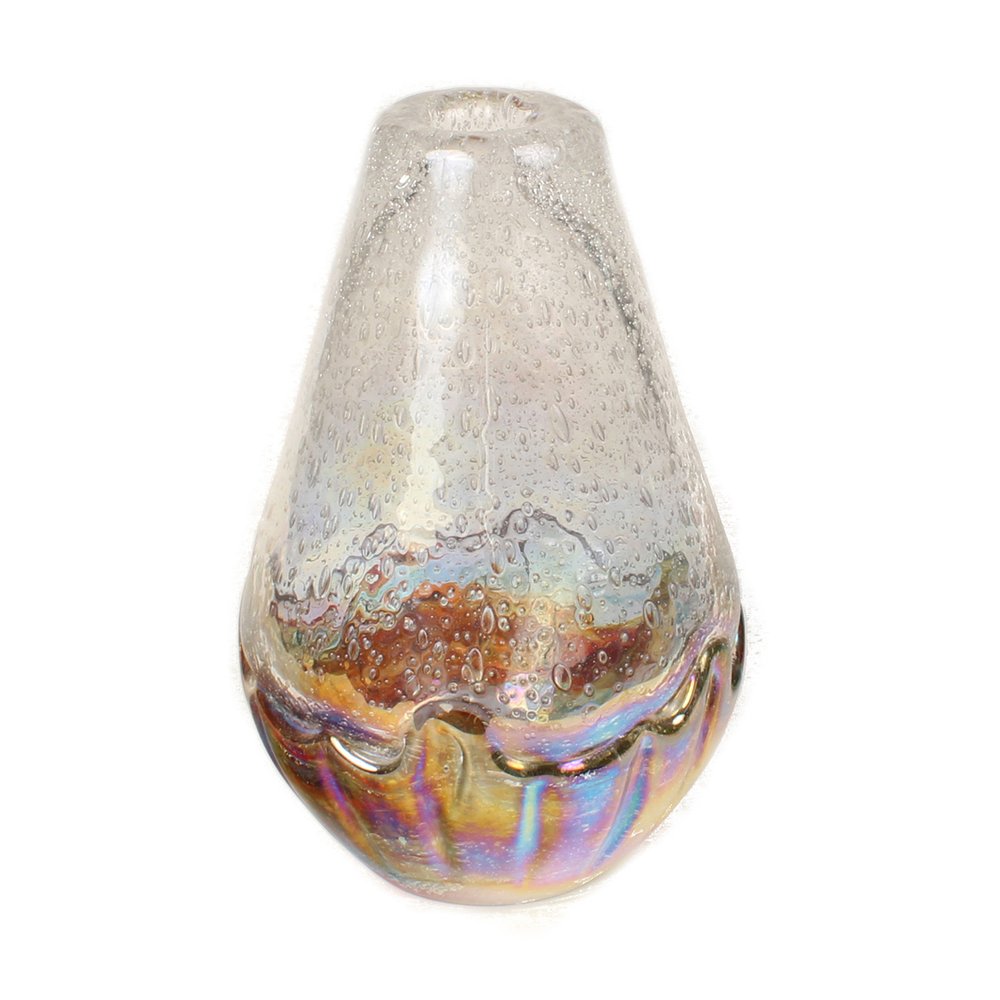This image depicts a teardrop-shaped blown glass object with a hole at the top, set against a white background. The object features a transition from clear glass at the top, which is embedded with small bubbles that descend about four-fifths of the way down, to a multicolored, reflective bottom. The bottom section showcases a rainbow-like glaze with hues of orange, purple, blue, and pink, exhibiting a metallic sheen that changes depending on the angle of light. The overall shape resembles a hurricane lamp piece or a decorative vase, with a rounded bottom that might evoke the shape of a Russian nesting doll. The glass appears thick, and there is a possibility of seeing through to the other side, adding a slight touch of gold and a light area down the middle, giving it a dynamic and reflective quality.